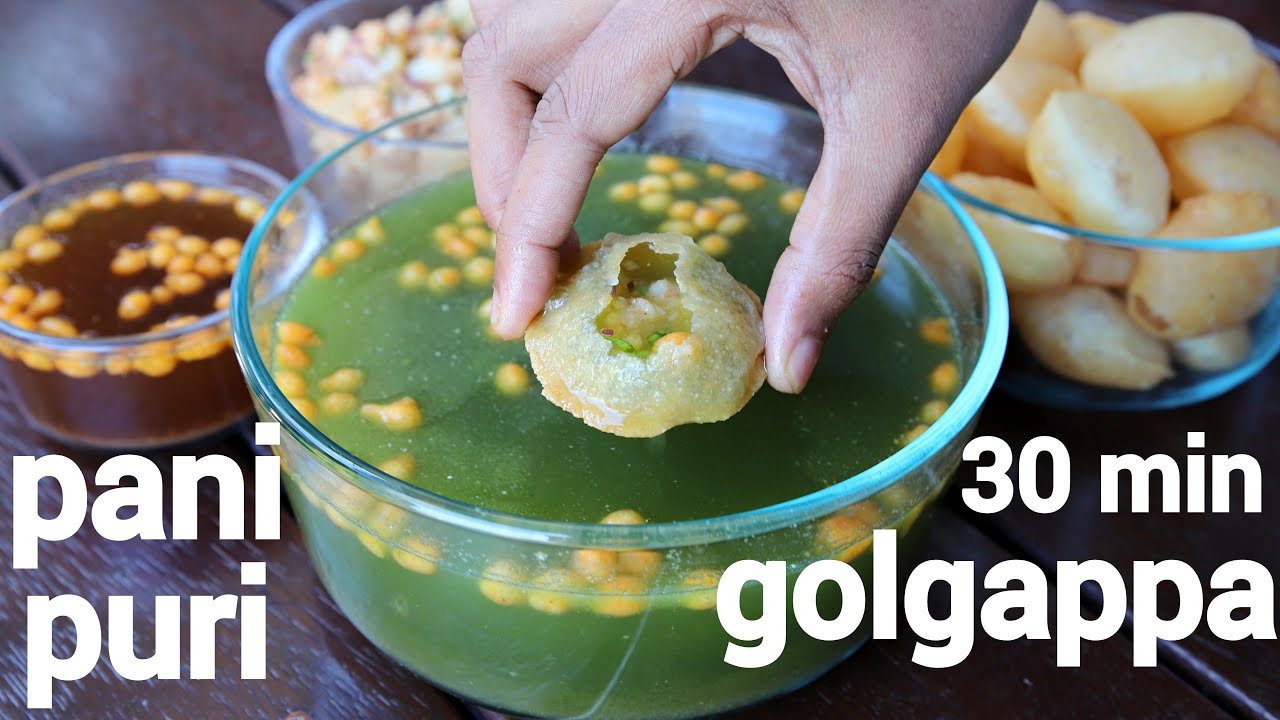The image captures a vibrant and detailed culinary scene likely derived from a video thumbnail. It prominently features white text on both sides: "Panipuri" on the left and "30-Minute Goal Gapa" on the right. Central to the image is a large, transparent glass bowl containing green liquid with yellow, corn-like pieces floating in it. A Caucasian hand descends from the top, dipping a fried, stuffed snack that appears to be partially broken open.

Surrounding this main bowl on a wooden table are several other glass bowls of varying sizes. To the right, there's a bowl filled with what look like fried pastries. On the left, one bowl holds a red liquid with similar corn-like pieces floating in it, and another bowl further back also appears to contain some variety of fried foods. The entire setup presents an array of colors with green, yellow, red, brown, and white hues, emphasizing the diverse and rich nature of the displayed foods.